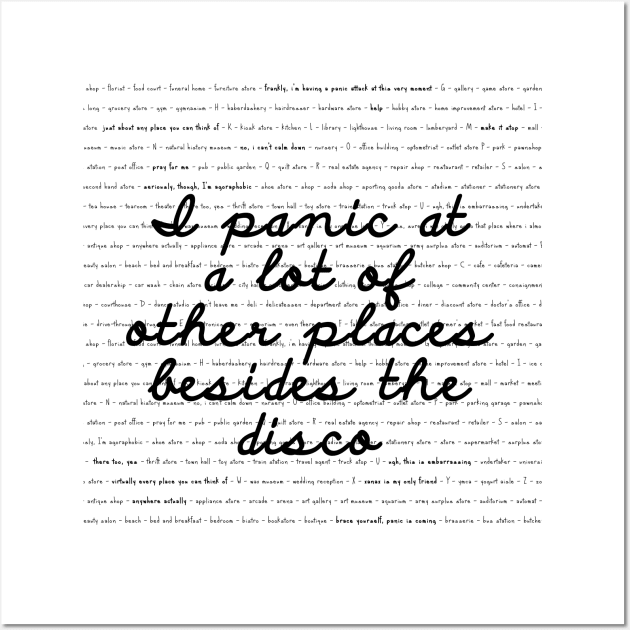This image features a digitally captured screenshot of a squared piece of paper filled with handwritten text in black cursive script. In the very center of the page, bordered by ample white space, is a prominent statement: "I panic at a lot of other places besides the disco." The central phrase is meticulously aligned to form a square shape. Surrounding this quote, the page is densely packed with uniform, small handwriting, interspersed with occasional bold words. Although the text is largely illegible due to its minute size, bits and pieces are discernible, mentioning places like florists, food courts, funeral homes, and furniture stores, and phrases such as "frankly, I'm having a panic attack at this very moment." The consistent black cursive writing, coupled with the intentionally bolded words throughout, reflects the individual's struggle with anxiety and panic attacks, giving a detailed and repetitive account of their experiences. The overall layout, devoid of any additional marks, emphasizes the overwhelming presence of text and the personal narrative it conveys.